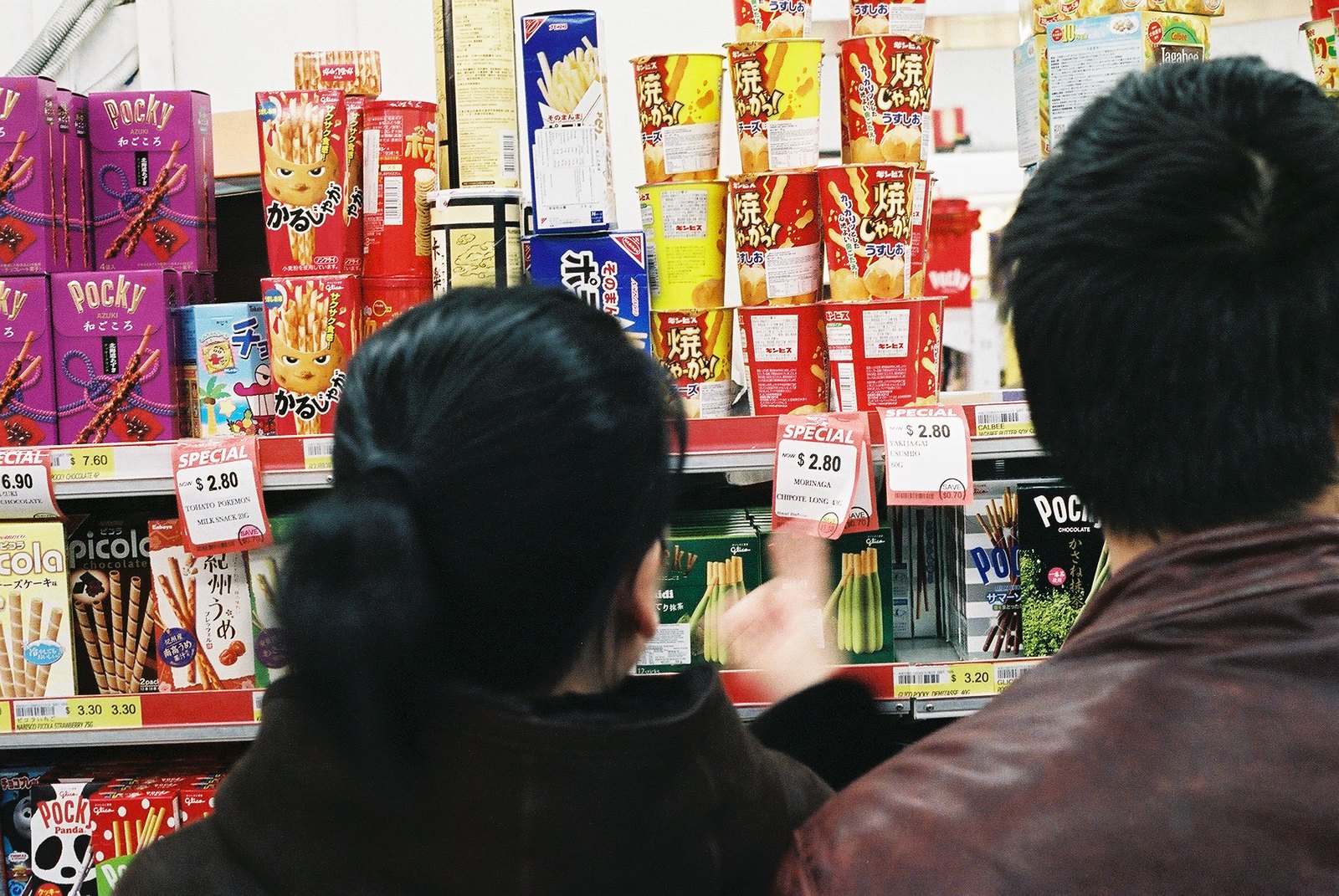In this photograph taken inside what appears to be an Asian grocery store, we see the partial back views of two people—a woman on the left and a man on the right—both intently browsing the brightly-colored snack section. The woman, identifiable by her long black hair pulled into a ponytail and her dark or black coat, stands next to the man who is sporting short black hair and a brown leather jacket. Both figures are only shown from the head down to a little below the shoulders, with the man's right side slightly cut out of the frame. They are focused on a shelf stocked with various treats, including Pocky and Piccolo, characterized by their vibrant packaging in purples, reds, and greens. Prominent red and white sale tags are visible, advertising specials such as $2.80 for certain items. Among these, specific signs read "special $6.90," "special $2.80," repeated multiple times. The scene captures a moment in which the couple seems captivated by the diverse range of snack offerings available in the store.